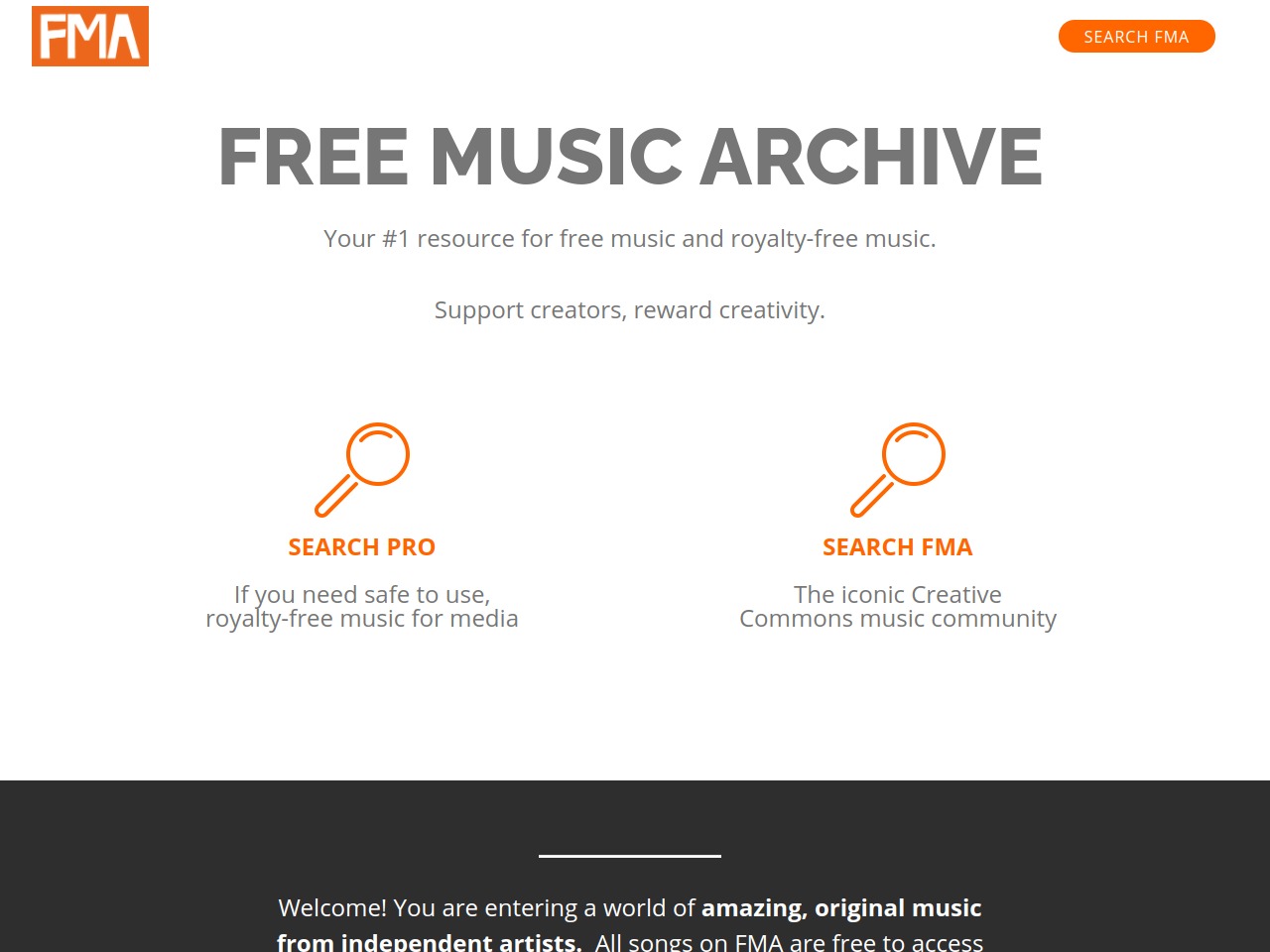This image is a desktop screenshot with ample white space. No web address, browser, or operating system details are visible. On the left side, there is an orange rectangle with "FMA" written in white letters. To the right, there is a rounded rectangular button, resembling a pill shape, with the text "Search FMA" in white.

Prominently displayed in bold gray text is the title "Free Music Archive." Below this, in smaller, unbolded text, it reads: "your number one resource for free music and royalty-free music. Support creators, reward creativity."

Underneath this description, two orange magnifying glass icons are positioned side by side. The left icon is accompanied by the text "search pro," with a note indicating it is for "safe to use royalty-free music for media." The right icon has the text "search FMA," indicating the "iconic Creative Commons music community."

Further down, a black rectangle with a white horizontal line in its center contains a welcoming message. The text reads: "Welcome, you are entering a world," with the phrase "amazing original music from independent artists" bolded. The message continues in regular text: "all songs on FMA are free to access."

This website appears to be a free music platform frequently utilized by creators for YouTube and TikTok videos.